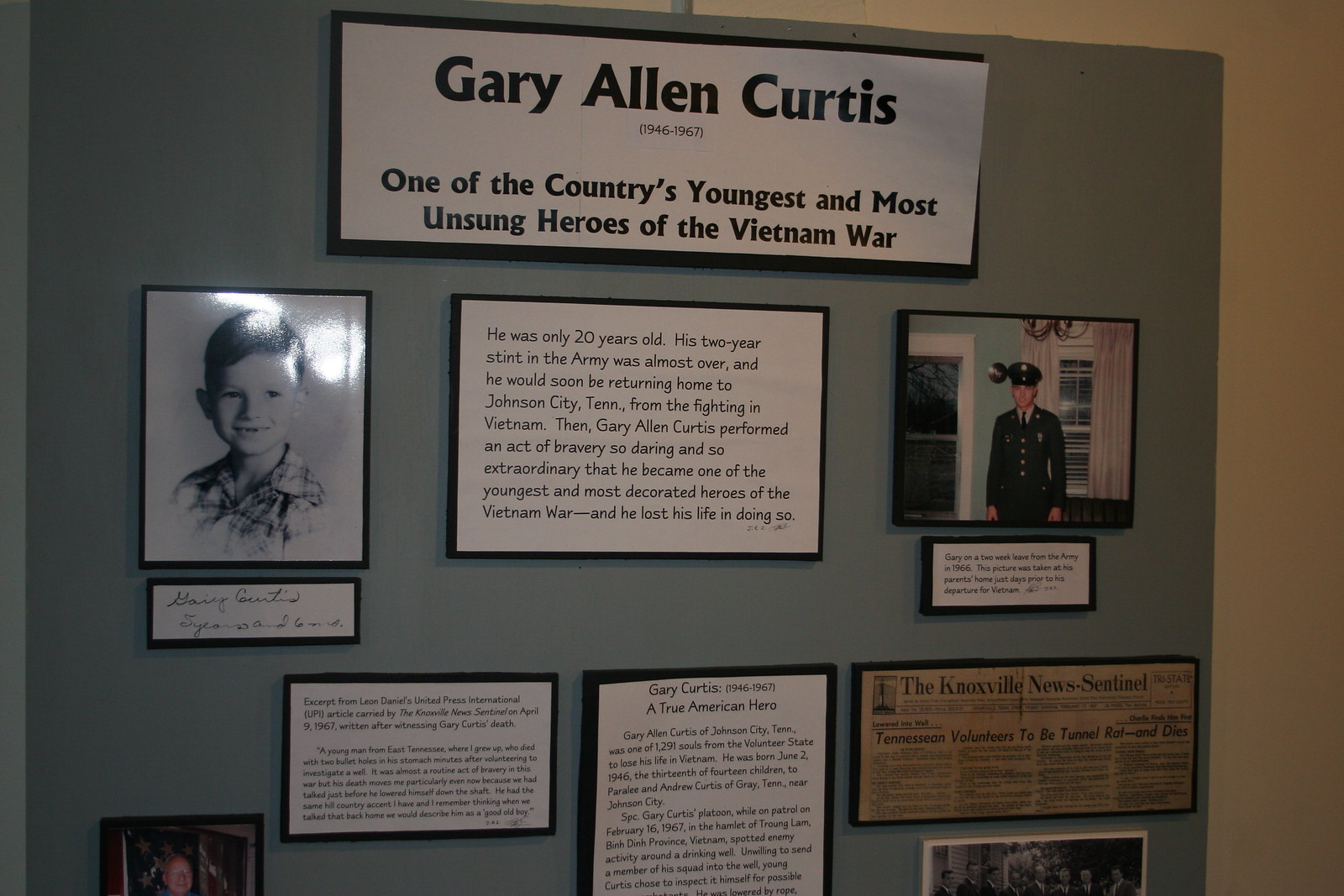The display is a detailed tribute to Gary Allen Curtis, featuring a collage of photographs, text, and newspaper clippings. At the top, in a horizontally oriented white rectangle with black text, it reads, “Gary Allen Curtis, 1946-1967, one of the country's youngest and most unsung heroes of the Vietnam War." The left side of the display features a black-and-white photograph of Curtis as a young boy, labeled in cursive as "Gary Curtis, five years old and six months." To the right of this, a text box narrates his story: "He was only 20 years old, his two-year stint in the Army was almost over, and he would soon be returning home to Johnson City, Tennessee from the fighting in Vietnam. Then, Gary Allen Curtis performed an act of bravery so daring and so extraordinary that he became one of the youngest and most decorated heroes of the Vietnam War, and he lost his life in doing so."

A larger photograph to the right shows Curtis in a green military uniform, against a blue background with what appears to be a window, a door, and a gold chandelier in the frame. Below all this, a cutout from the "Knoxville News Sentinel" newspaper highlights a bold headline: "Tennessean volunteers to be tunnel rat and dies." The display combines various elements to honor the bravery and sacrifice of Gary Allen Curtis, painting a vivid picture of his short yet heroic life.